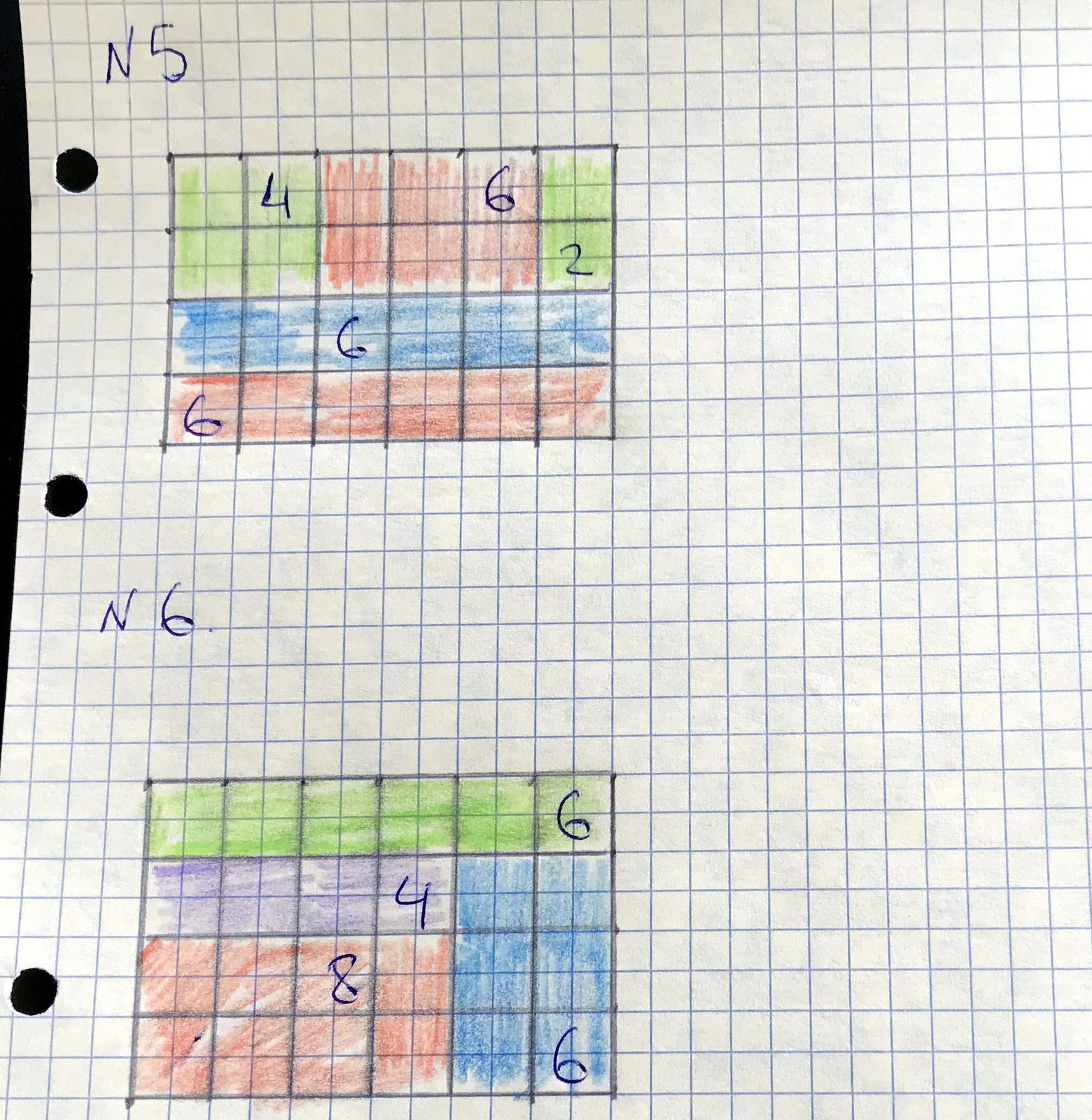In this image, a piece of graph paper fills the frame, primarily occupying the center and right portion while a sliver of black appears on the left-hand side through three holes punched along its margin. The white paper, decorated with an intricate grid of small squares formed by blue lines, seems to serve as the backdrop for a detailed mathematical illustration or homework assignment.

At the top-left corner, just above the highest hole, is inscribed "N5" in blue ink. Below this notation lies a meticulously drawn graph, composed of a rectangle spanning four squares in height and six in width. The top row of this grid is colored as follows: green, green, red, red, red, green. Each square is filled with its respective color. The second row mirrors the first in its color arrangement. The following two rows deviate, with the third row entirely blue and the fourth row entirely red.

Within these colored squares, several numbers are penned in blue ink. In the first block of the second row, the number "4" is written. The fifth box of the same row contains the number "6", while the sixth box holds the number "2". In the next row, the third box is numbered "6", and in the final row, the first square is marked with a "6".

A few lines below this grid, the designation "N6" is penned in blue ink, introducing another four-by-six grid. This second square grid features a different color pattern: the first row is consistently green, with the number "6" in the last block. The second row comprises four purple squares followed by a block with the number "4" and a final pair of blue squares. The third row includes four red squares, with the third box numbered "8", and is concluded with two blue squares. The last row mirrors the color pattern of the third row and concludes with the final blue square numbered "6". All numbers throughout the grid are carefully inscribed in blue ink, indicative of the precise and methodical nature of the mathematical documentation.